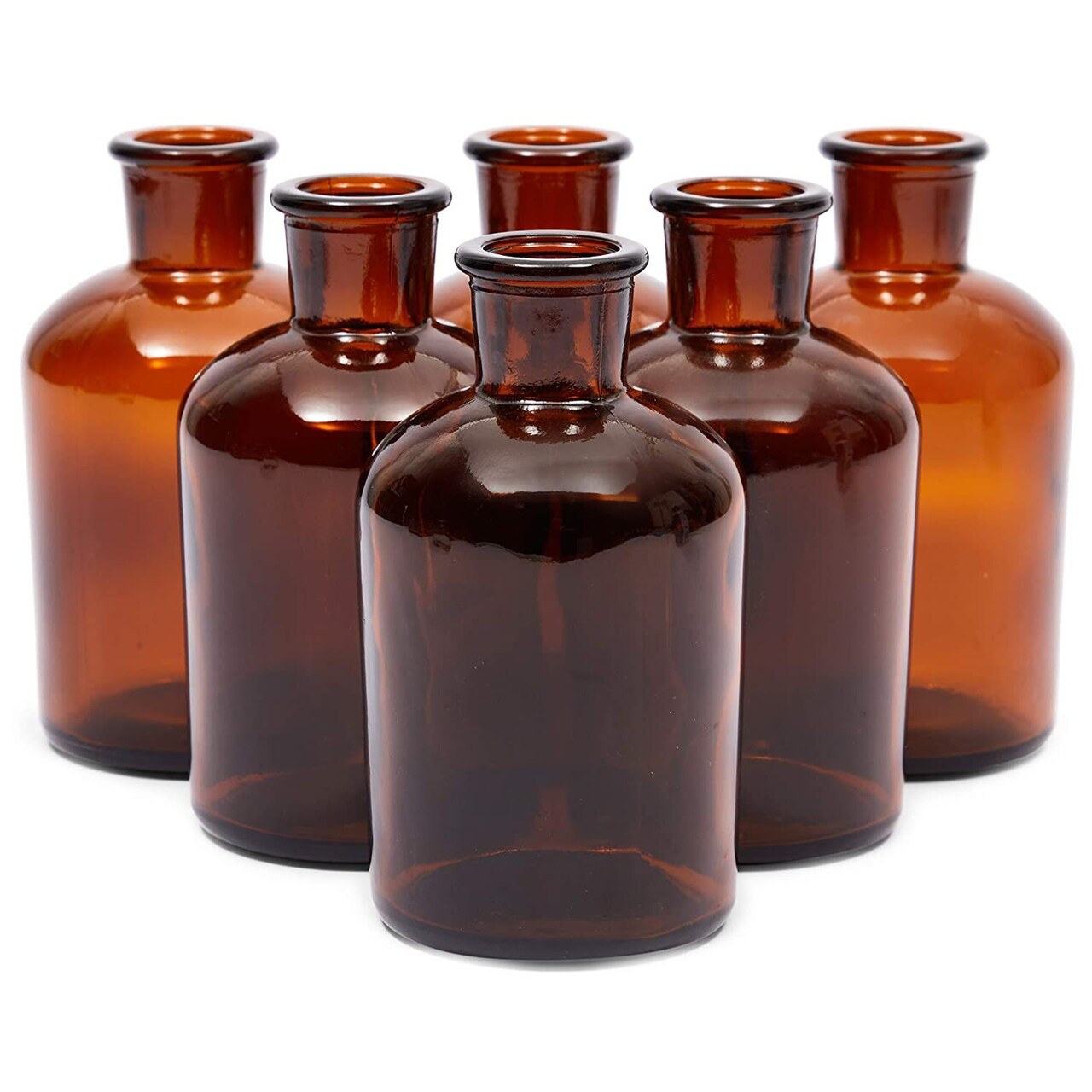This is a rectangular color photograph featuring six cylindrical glass bottles arranged in a triangular formation against a solid white background. In the foreground, there is a single dark amber bottle. Behind it, there are two bottles of the same dark amber shade. The final row consists of three lighter amber bottles. All the bottles share a glossy finish that reflects ceiling lights, and they taper into a skinnier top section with a wide brim that transitions smoothly into a dome shape. The bottles are empty, uncapped, and have no visible writing or markings. There are no other elements such as people, animals, buildings, or vehicles in the image.